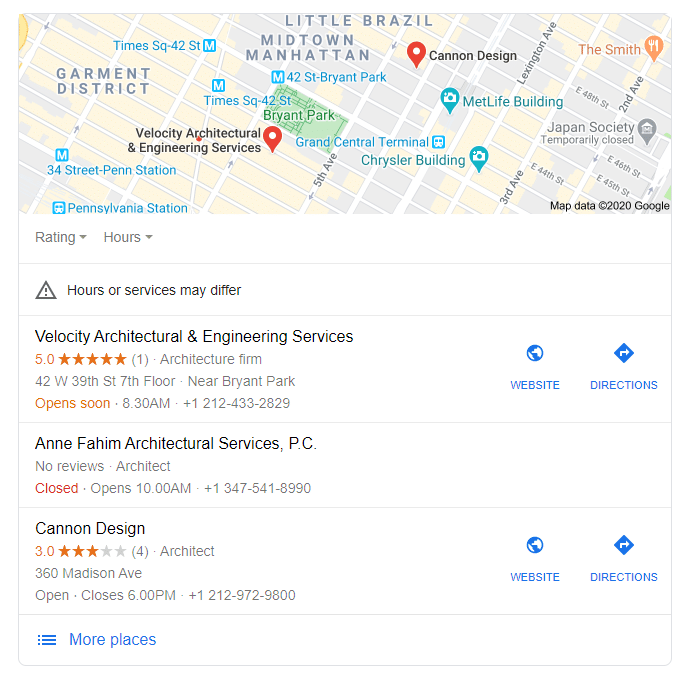The image displays a Google search results page featuring a map with location pins for "Velocity Architectural Engineering Services" and "Canon Design" in Midtown Manhattan. At the top of the map, there are drop-down menus labeled "Rating" and "Hours," followed by a warning triangle with an exclamation mark indicating that "Hours or services may differ." 

Below the map, "Velocity Architectural Engineering Services" is listed with a five-star rating based on one review. The firm's address is "42 West 39th Street, 7th Floor, near Bryant Park," and it is noted to open soon at 8:30 AM. The contact number given is +1 212-433-2829, with hyperlinks to their website and directions.

Following this, "Ann Fahim Architectural Services, PC" is listed with no reviews. It is described as being closed currently but will open at 10 AM. The provided contact number is +1 347-541-8990.